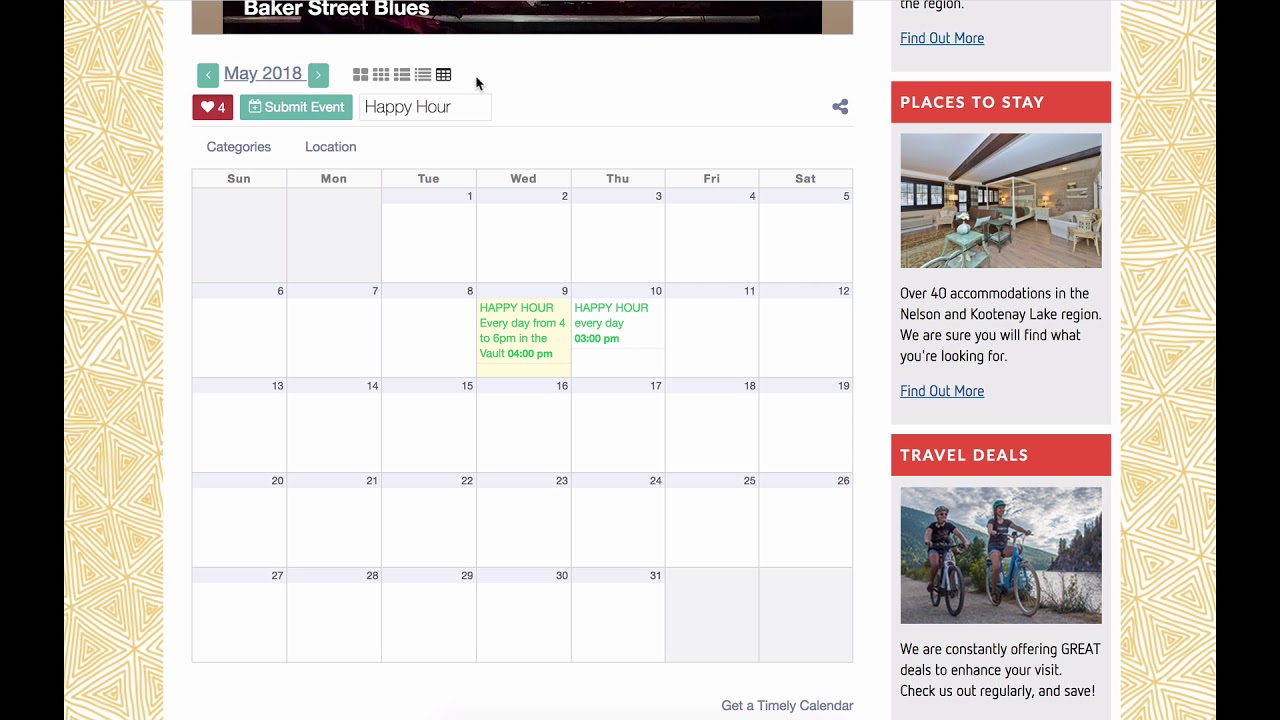The image showcases a calendar titled "Baker Street Blues" dated May 2018, featuring both English and Asian text. The calendar layout begins with May 1st, a Tuesday, and concludes on Thursday, May 31st. Notable entries include “Happy Hour” on the 9th and 10th, highlighted in green text, with the 9th also shaded in a manila hue.

The design includes a distinct yellow patterned border on the left side, mirrored by a black border on the right. Additionally, the calendar features two informative sections: “Places to Stay” and “Travel Deals.” The "Places to Stay" section lists over 40 accommodations in the Nelson and Kulene Lake region. The "Travel Deals" section provides details on various offers. Both sections include interactive "Find Out More" links for additional information.

The right-hand side background matches the left, with a yellow and black design. The overall theme blends organized event planning with travel and accommodation information, presented in a visually appealing and functional layout.